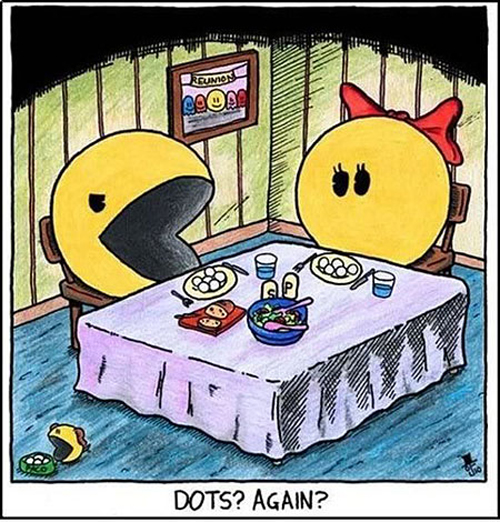The image is a detailed cartoon comic strip featuring Pac-Man and Mrs. Pac-Man sitting at a dining room table covered by a light purple tablecloth. The table is set with a red breadboard holding sliced bread, a blue bowl of salad, salt and pepper shakers, two glasses of water, and individual plates in front of Pac-Man and Mrs. Pac-Man, each holding small white dots. This is humorously underscored by Pac-Man's exclamation, "Dots again," referencing his iconic game habit of eating dots. The scene is enriched with a yellow wall background, adorned by a reunion photograph depicting Pac-Man with blue, orange, pink, and red ghosts, purportedly from Pac-Man’s high school days. At the bottom left corner, a small dog Pac-Man, named Paco, is shown eating from a green food bowl, with an artist’s mark appearing in the bottom right corner.